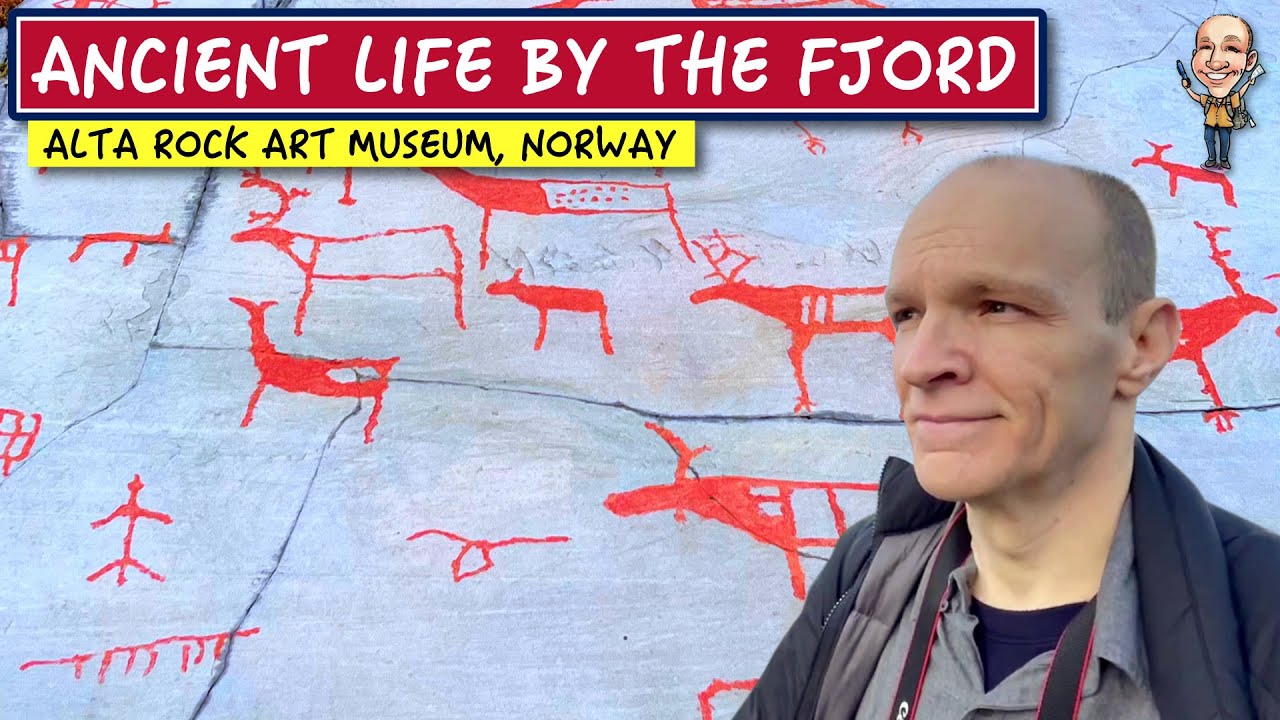The image showcases a horizontal, rectangular photograph of an older, bald man with pale skin. He stands in front of a concrete sidewalk marked with red stick-figure drawings, resembling reindeer and moose, evoking ancient cave art. The sidewalk is gray with visible cracks. The man is wearing a blue jacket and a gray collared shirt, with a black strap hanging around his neck. Prominently displayed above his head in the top left corner, a red rectangle features white text reading "Ancient Life by the Fjord". Directly beneath it, a yellow rectangle with black text announces "Alta Rock Art Museum, Norway". The artwork and text elements combine to create a visually engaging narrative of historical and cultural intrigue at the museum.